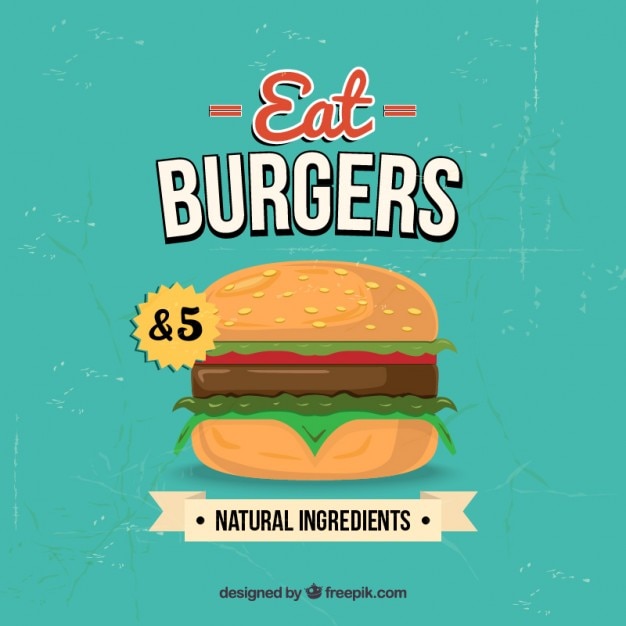The image is a computer-animated advertisement for burgers, featuring a detailed illustration of a classic cheeseburger on a light blue background with white speckles for added texture. At the top, in red letters with white outlines and resembling an equal sign, it says "EAT," followed by the word "BURGERS" in bold white letters with a black outline. Below the text, the cheeseburger illustration includes a sesame-seeded top bun, layers of lettuce, red tomato, a juicy patty, green sauce, and melting cheese. Beneath the burger, a white banner with black text declares "NATURAL INGREDIENTS," and next to it is the notation "$5" alongside the text "Designed by Freepik."